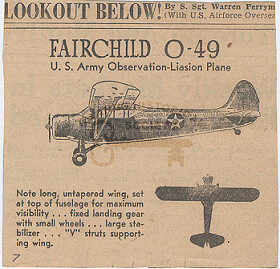This is an old newspaper feature, showcasing the Fairchild O-49 U.S. Army Observation Liaison Plane, attributed to S. Sergeant Warren Perry. The article is titled "Look Out Below!" in bold black letters and is likely dated back to the 1930s. The image has a vintage feel, illustrated in black-and-white ink. It includes two sketches of the aircraft: a detailed side view and a shadowed top-down view. Key features of the plane, noted in the article, include long untapered wings set atop the fuselage for maximum visibility, fixed landing gear with small wheels, a large stabilizer, and V-struts supporting the wing. The U.S. Air Force logo is visible on the plane, reinforcing its historical military significance. The number 7 appears in the lower left-hand corner of the image.